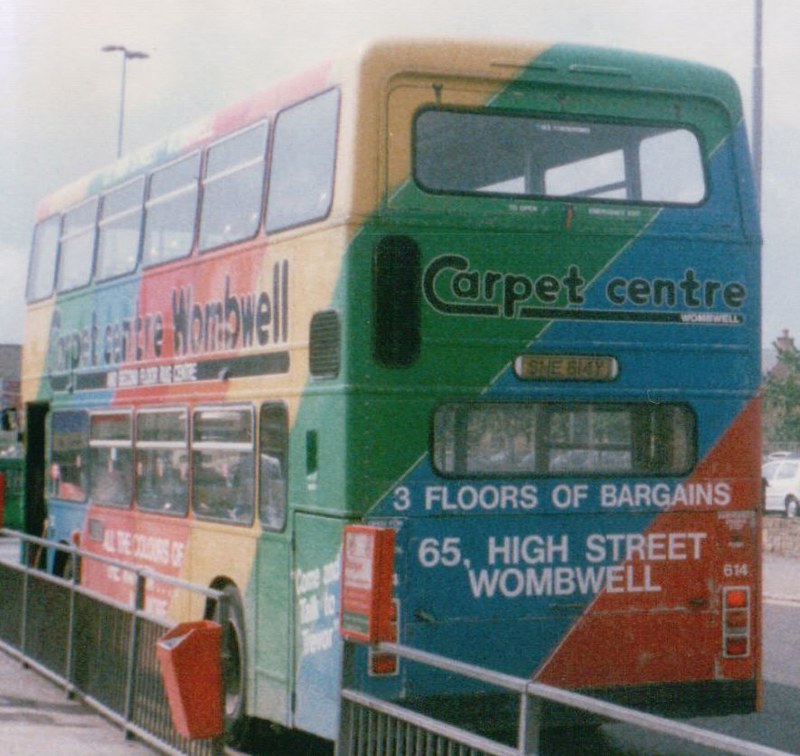This photograph features a vibrant, double-decker tour bus, prominently adorned with a diverse palette of colors including red, blue, green, yellow, gray, orange, black, and white. Identified as bus number 614, the vehicle boasts the name “Carpet Center” and is emblazoned with promotional text stating, "Three Floors of Bargains, 65 High Street, Wombwell." The bus displays a license plate reading SNE614Y.

The bus itself is depicted at an angle, with the camera primarily capturing the rear and part of the side. The lower portion of the bus includes five windows on the side, while the upper deck has six windows. The rear view reveals two windows – one on the top deck and one on the bottom. Additional text on the bus reads, "Come and talk to Trevor," although some sections are rendered blurry and less readable.

The setting is outdoors, adjacent to a wooden fence and a guardrail, suggesting the bus may be parked near a bus station. Poles are visible in the background, and the bus occupies most of the image, emphasizing its colorful and eye-catching design.